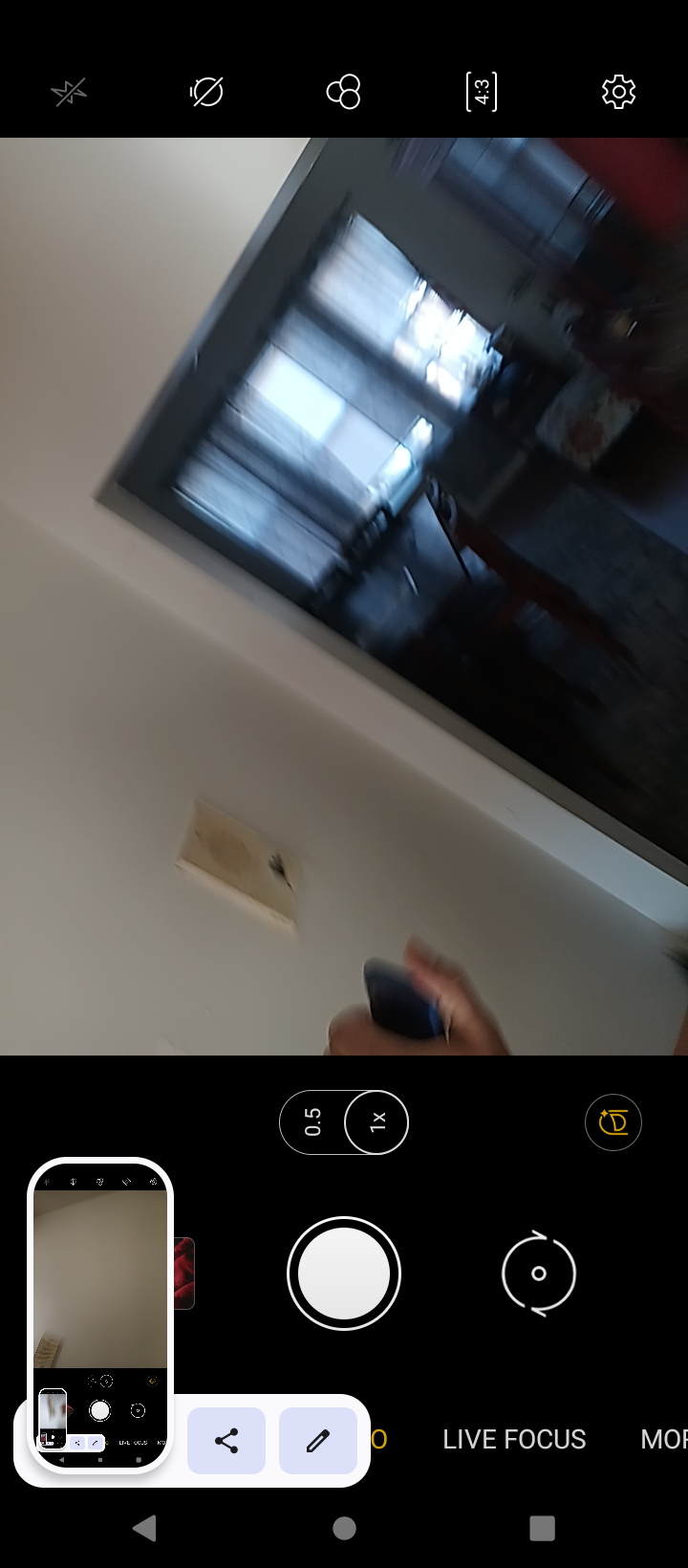In this color screenshot taken from a mobile device, the camera app is open, capturing a video inside a house. The image showcases a scene through a slightly angled perspective, leading to a white doorway opening into a dining room. The room features white walls, a window in the background with curtains, and a partially seen wooden dining table with chairs around it; a cabinet is also faintly discernible on the right-hand side. The central image is somewhat blurred but includes a left hand holding a black object. Across the bottom of the screenshot, typical camera app controls are visible, including options like "Live Focus." The screenshot appears to be taken from an Android phone, highlighted by multiple layers of screenshots framing the camera app interface.